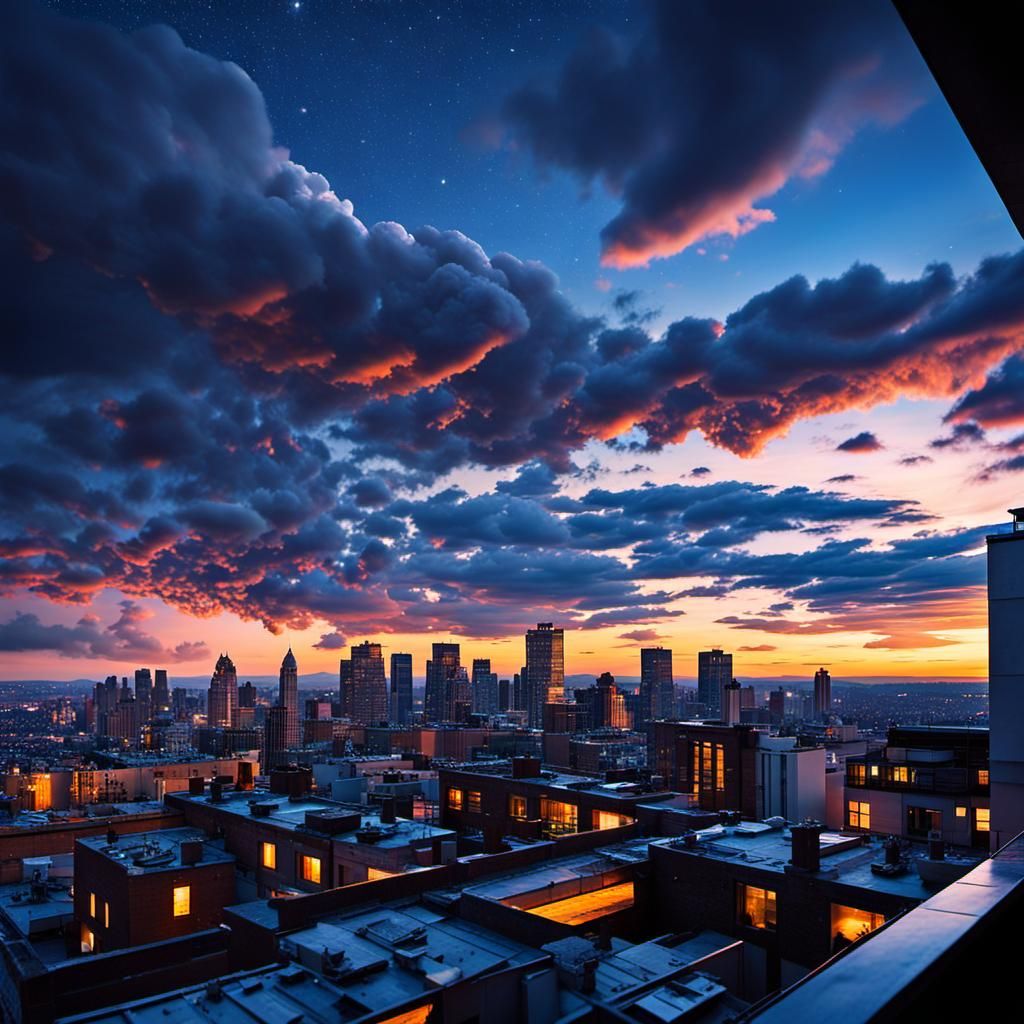The image showcases a digitally-rendered, almost photo-realistic cityscape from a high vantage point, possibly a balcony. The scene captures a sprawling downtown area transitioning into night, with a richly detailed sky and vibrant city lights. Thick dark gray clouds with orange and pink hues dominate the sky, interspersed with glimpses of stars and a distant golden glow, suggesting a recent sunset. Skyscrapers rise prominently in the center of the image, flanked by an array of smaller, rectangular apartment buildings and residential districts, all illuminated by warm, candelabra-like glows from countless windows. The buildings exhibit various shapes and sizes, some tall and cylindrical, others shorter and square, and numerous metal objects can be observed perched on their roofs. The skyline stretches out in a harmonious blend of architectural forms and twinkling lights, evoking the bustling essence of an evening cityscape.